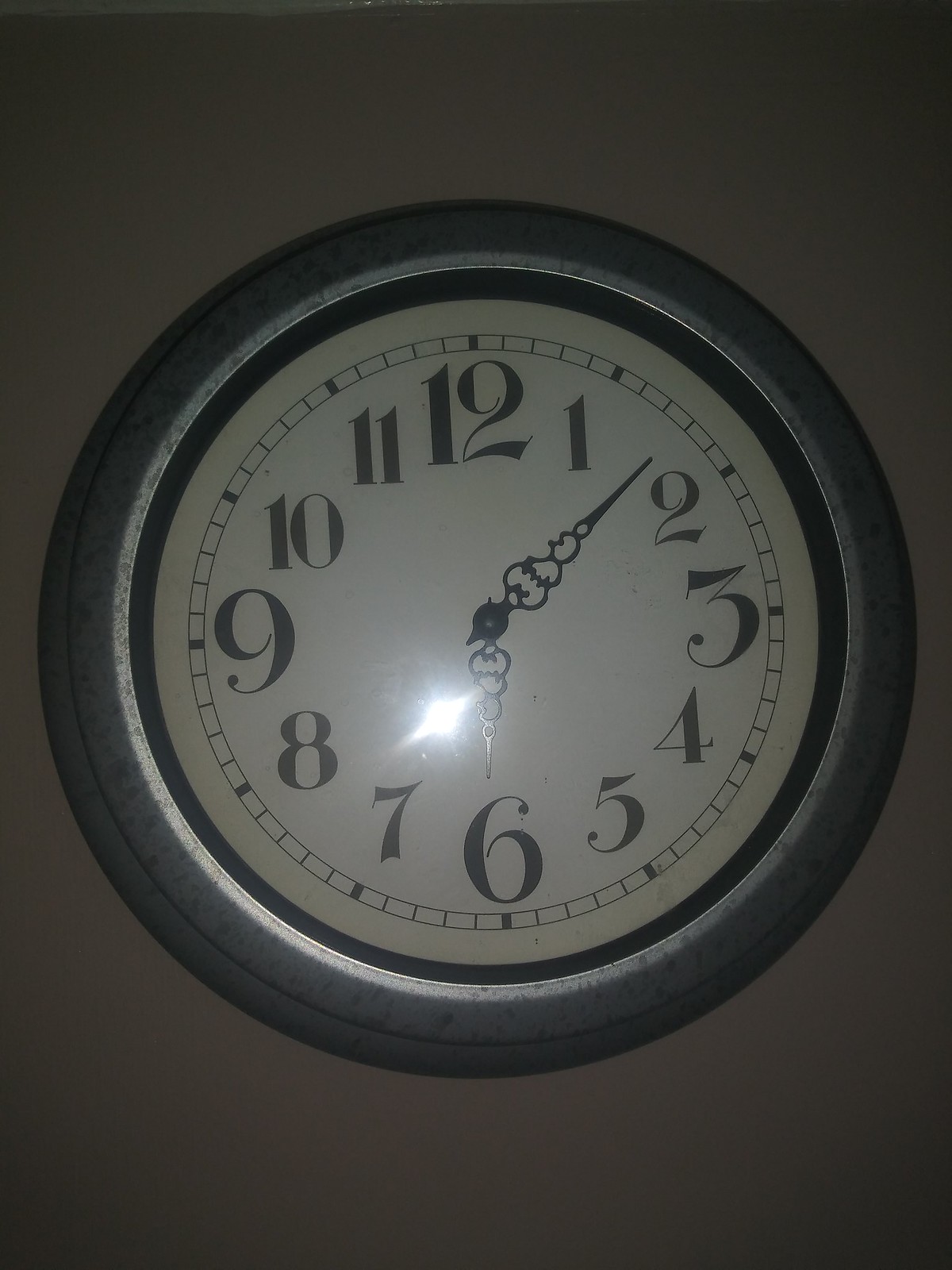The image is a portrait-oriented photograph featuring a wall clock. The background appears dark gray, likely due to poor lighting, with the corners being darker than the central area around the clock. The clock itself is circular and mounted against the wall, raised slightly to give it a three-dimensional, Frisbee-like appearance. The clock's outer rim is a silvery gray, enclosing an inner black circle which frames the clock face.

The clock face has a white background with standard numerals ranging from one to twelve. The numerals at twelve, three, six, and nine are significantly larger and more prominent than the others and have a curvy, less formal design in a dark gray shade instead of pure black. The clock hands are ornate, with intricate, circular designs along their lengths. The hour hand points slightly to the left of the six, while the minute hand indicates eight minutes past the hour, making the time displayed 6:08. A shiny, reflective area is visible to the left of the hour hand, likely from the camera flash.